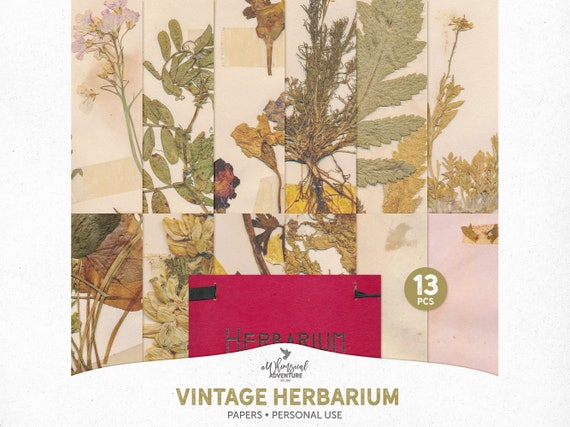This product photograph showcases the packaging for a 13-piece set of printed papers, set against a white background. The front of the packaging features thumbnail images of each paper, all adorned with various floral and leaf designs, including pink flowers, green leaves, dried flowers, and yellow flowers, giving a vintage pressed flower aesthetic. The patterns are displayed on a pink backdrop, framed by a white border on the left, right, and bottom edges. At the bottom, bold gold text spells out "VINTAGE HERBARIUM" with "PAPERS, PERSONAL USE" written beneath in black. Above the text, there's a logo or watermark of the company. On the bottom right corner, a gold circle with white text indicates "13 Pieces." Additionally, a small, rectangular pink sign labeled “herbarium" is tucked beneath several of the paper images.